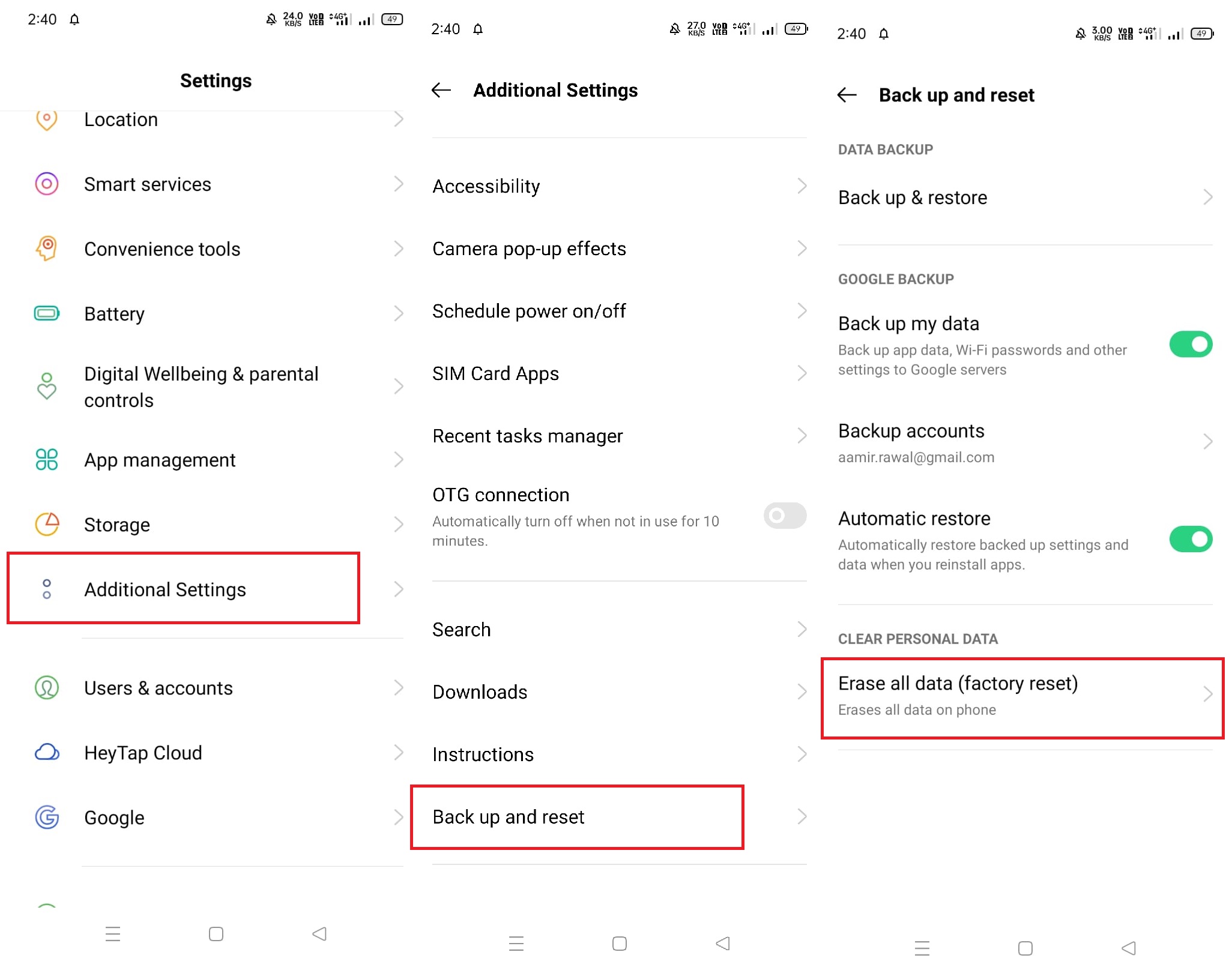The image is a sequence of three mobile device screenshots, meticulously captured and annotated. 

- **First Screenshot:**
  - **Top Bar:** The time shows 2:40 PM, battery life at 49%, and various data icons are visible.
  - **Settings Page:** Displayed are the menu options: Location, Smart Services, Convenience Tools, Battery, Digital Well-being and Parental Controls, App Management, Storage, Additional Settings, Users and Accounts, HeyTap Cloud, and Google.
  - **Highlight:** A red box is drawn around the "Additional Settings" icon.

- **Second Screenshot:**
  - This screenshot expands the "Additional Settings" menu to reveal its options: Accessibility, Camera Pop-up Effects, Schedule Power On/Off, SIM Cards and Apps, Recent Task Manager, OTG Connection, Automatically Turn Off When Not In Use For 10 Minutes, Search, Download Instructions, and Backup and Reset.
  - **Highlight:** A red box surrounds the "Backup and Reset" option.

- **Third Screenshot:**
  - This screenshot dives into the "Backup and Reset" menu:
    - **Menu Options:** Data Backup, Backup and Reset, Google Backup.
    - **Backup My Data:** An option to back up app data, Wi-Fi passwords, and other settings to Google servers, toggled on.
    - **Backup Account:** Listed as aamir.rawal.com.
    - **Automatic Restore:** An option to automatically restore backed-up settings and data when apps are reinstalled, toggled on.
    - **Clear Personal Data:** The "Erase All Data (Factory Reset)" option, highlighted with a red box.

The sequence visually guides the user through the process of accessing factory reset options within the mobile settings.